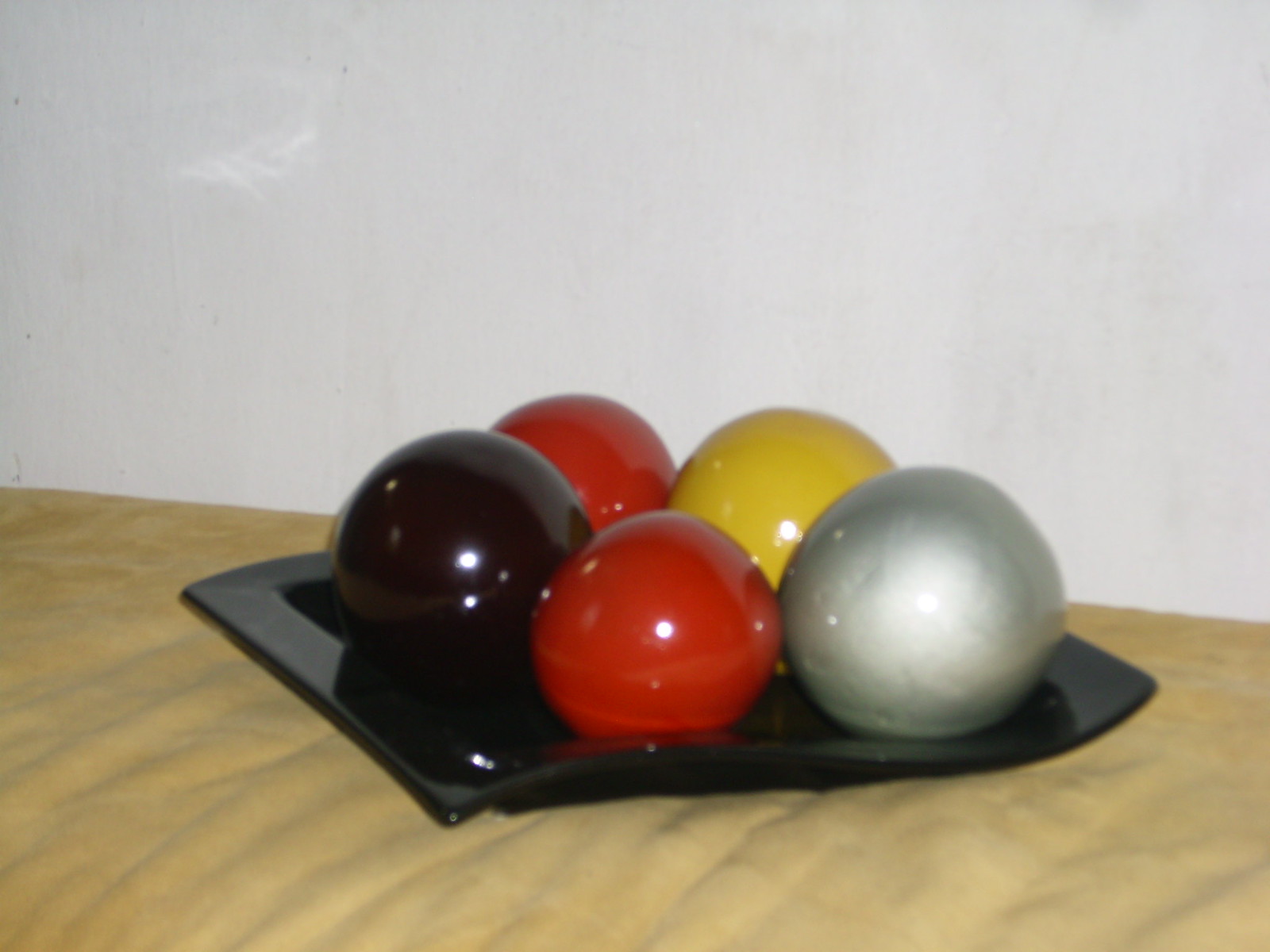The image depicts an arrangement of five reflective spheres on a wooden table with wavy lines in its texture. The wooden table, featuring a black holder or shallow bowl, stands before a plain white wall. The bowl contains two red balls, a yellow ball, a silver ball, and a darkish purple (or possibly black) ball. All the spheres are closely arranged, with light reflecting off their surfaces, adding a gleaming effect. The reflective black bowl holds the balls, which are described to be about the size of bowling balls, enhancing the artistic and striking quality of the composition.